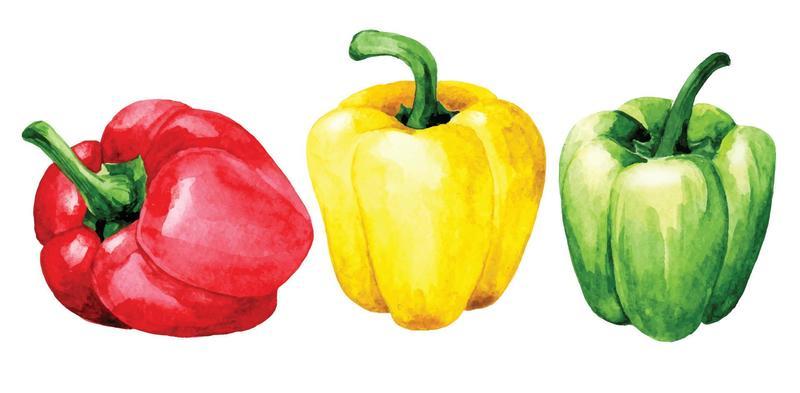This image features an illustrated watercolor drawing of three bell peppers arranged in a line against a white background. Each pepper has a realistic, glossy appearance. The bell pepper on the left is a deep red, lying on its side with a long, green stem and a slight shine. The central bell pepper is yellow, standing upright with a curved green stem and slight browning at the bottom. The pepper on the right is a solid green color, also standing upright. The green pepper shows a gradient with lighter sides, a darker top, and an even darker stem. All three peppers appear similar in size and exhibit meticulous details that highlight their natural look and vibrant colors.